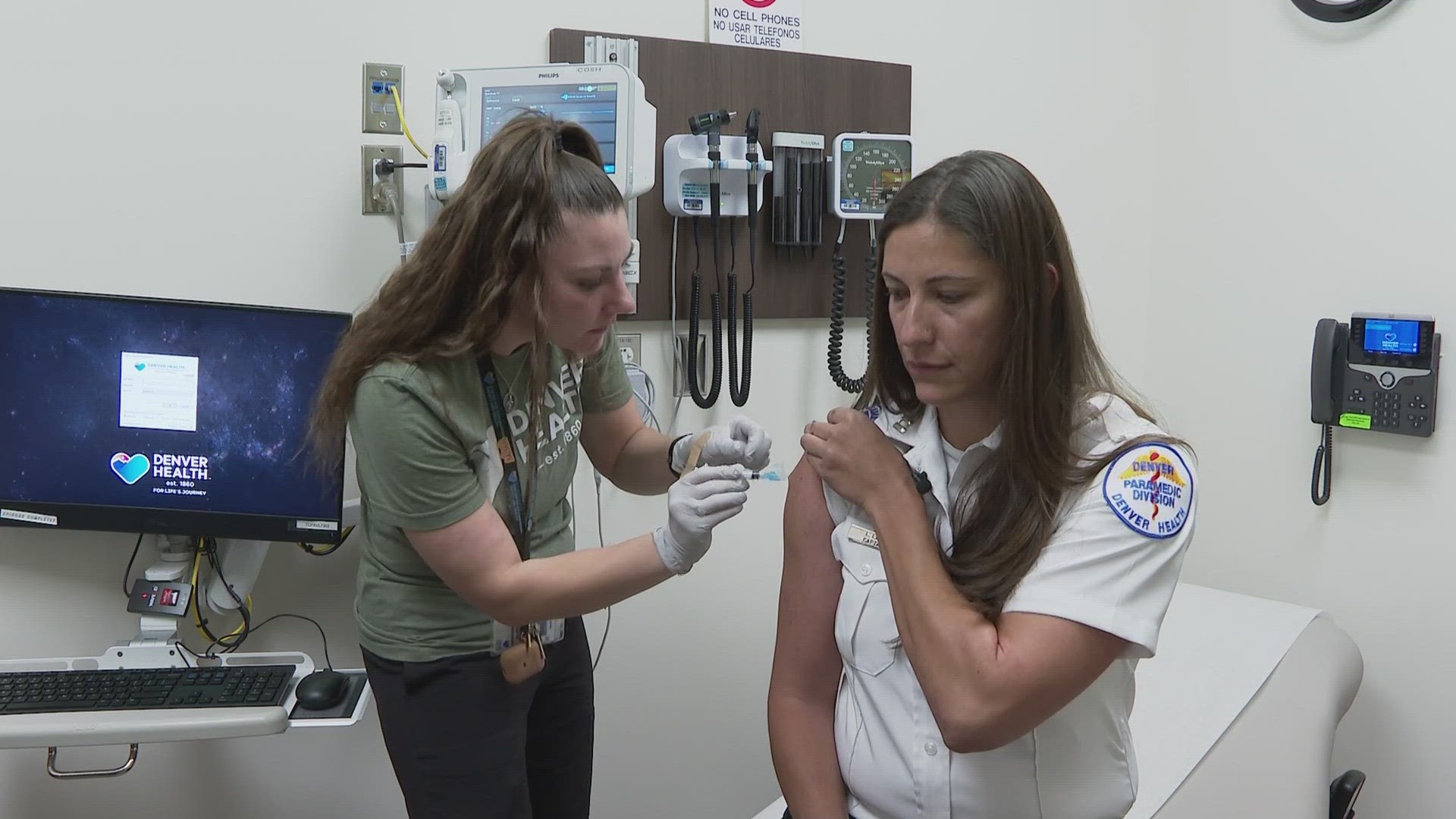The photograph captures a moment inside a Denver Health doctor's office, depicting a nurse administering a vaccine to a female paramedic. The patient is seated on an examination chair with her left sleeve rolled up, revealing a badge on her white button-up shirt that identifies her as a paramedic. The nurse, dressed in a light green shirt, black pants, and a lanyard with an ID tag, is focused on delivering the shot to the patient's upper arm. The room is equipped with various medical apparatus, including a blood pressure cuff and a computer setup to the left of the patient that displays "Denver Health" on the screen. Also visible are a wired telephone mounted on the wall and other typical medical equipment, creating a setting that is clearly within the treatment area of a medical facility.